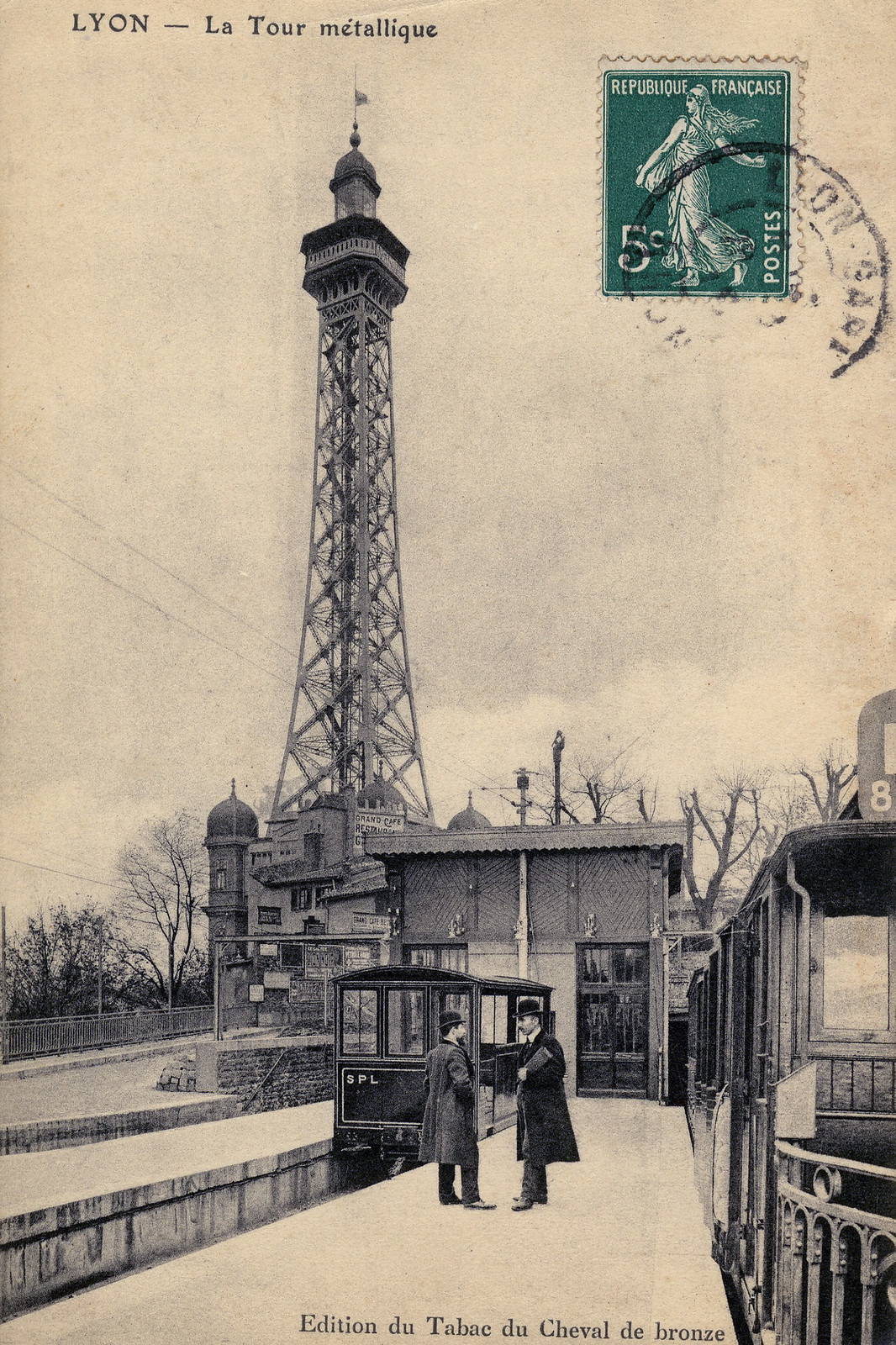This is a meticulously detailed color photograph of an old black-and-white postcard from Lyon, France. The top right corner features a green 5-cent stamp with the inscription "POSTES - Republic Francaise" and a postmark. At the top of the postcard, the caption reads "Lyon, La Tour Metallique," identifying the location and notable landmark. The image prominently displays the La Tour Metallique in the background, a towering metal structure with an observation deck at its peak, reminiscent of the Eiffel Tower. In the foreground, two men in early 20th-century attire stand on an outdoor platform, seemingly engaged in conversation, flanked by a train car or trolley on the right. A small station house is visible behind them, alongside scattered trees, but no other buildings are in sight. The bottom edge of the postcard bears the text "Édition de T-A-B-A-C de Cheval de Bronze," marking the publisher. The overall tone of the photograph is grayish-white, contributing to a sepia-toned, faded appearance that underscores the postcard's vintage charm.